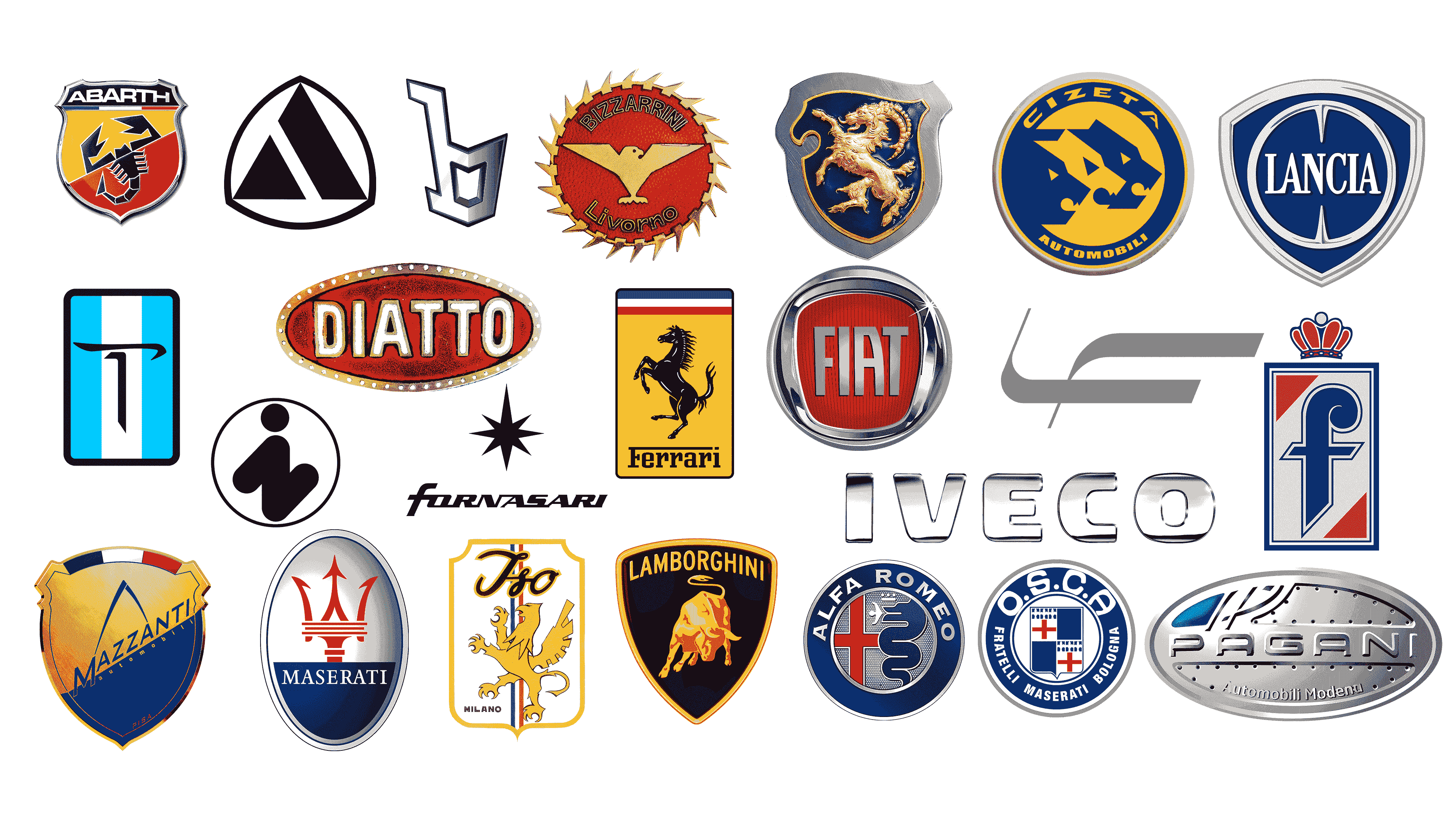The image displays a vibrant and detailed collection of 23 car brand logos, all of which are Italian. Each logo is distinctly designed and colored, set against a clean white background. Notable logos include Abarth's scorpion on a yellow-red shield, Alfa Romeo's serpent and red cross on a blue background, Diato's text on a brown oval, and Ferrari's iconic prancing horse on a yellow field. Fiat's badge shows its name in bold, capital letters with a red hue. Fornasari is signified by a simple black star, while Iveco stands out with its bold, capital text. Among other recognizable brands are Lamborghini, Maserati, Lancia, and Pagani, each logo featuring unique elements like animals, crowns, and stylized letters. The image is brightly lit and the clarity is excellent, making each logo's intricate design and color scheme easily observable.